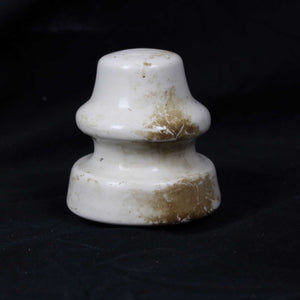The image displays an object against a black backdrop, resembling an old insulator used for connecting power lines. Made from a hard, glass-like material possibly confused for ceramic or granite, the object predominantly features a white color at the top. Its flat top angles down and flares out, akin to a hat or mushroom head, with a cylindrical middle section perfect for wrapping a wire around securely. The object, reminiscent of a pawn chess piece, has a thicker base that adds to its sturdy appearance. Additionally, there is notable browning or wear on one side, suggesting age or usage over time.